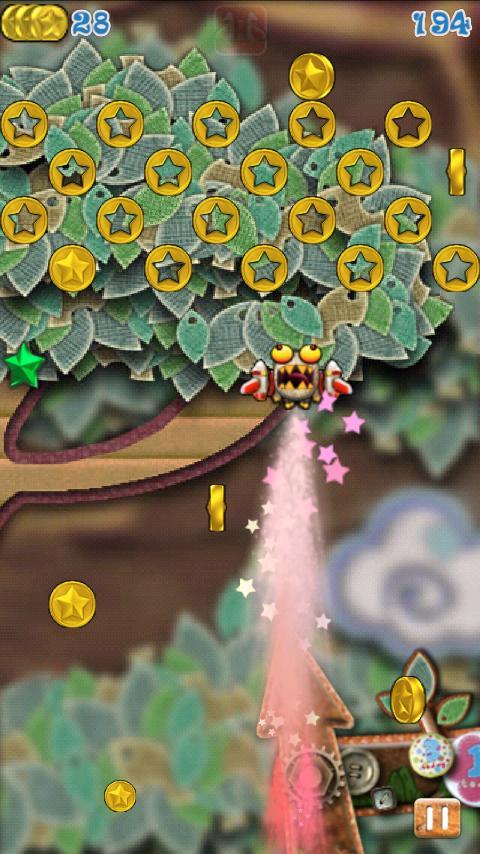Displayed is a vertically oriented rectangular scene resembling a screenshot from a video game. The background is artistically blurred, suggesting depth and focus on the foreground elements, with hints of brown and green foliage, and swirls of white and blue shapes. In the upper left corner, there's a cluster of gold coins with the number "28" displayed in blue text. On the upper right side, the number "194" is prominently featured in blue text outlined in white.

A stylized, whimsical tree dominates the center of the image. The tree has an exaggerated, video game-esque appearance, with brown outline branches and abundant green leaves, which vary in shade for a dimensional effect. Encrusted among the leaves are star-shaped coins.

At the base of the tree, a quirky, fish-like creature with bulging eyes and an open mouth displaying sharp teeth gazes upward. Adorning its side are laser-like details, and it seems to be emitting pink, sparkling fairy dust that includes tiny stars. Additional coins appear to be floating towards the blurred foliage below.

Towards the bottom of the image is a treasure chest, seemingly the destination for the falling items. Adjacent to the chest is a pause button, indicating active gameplay.